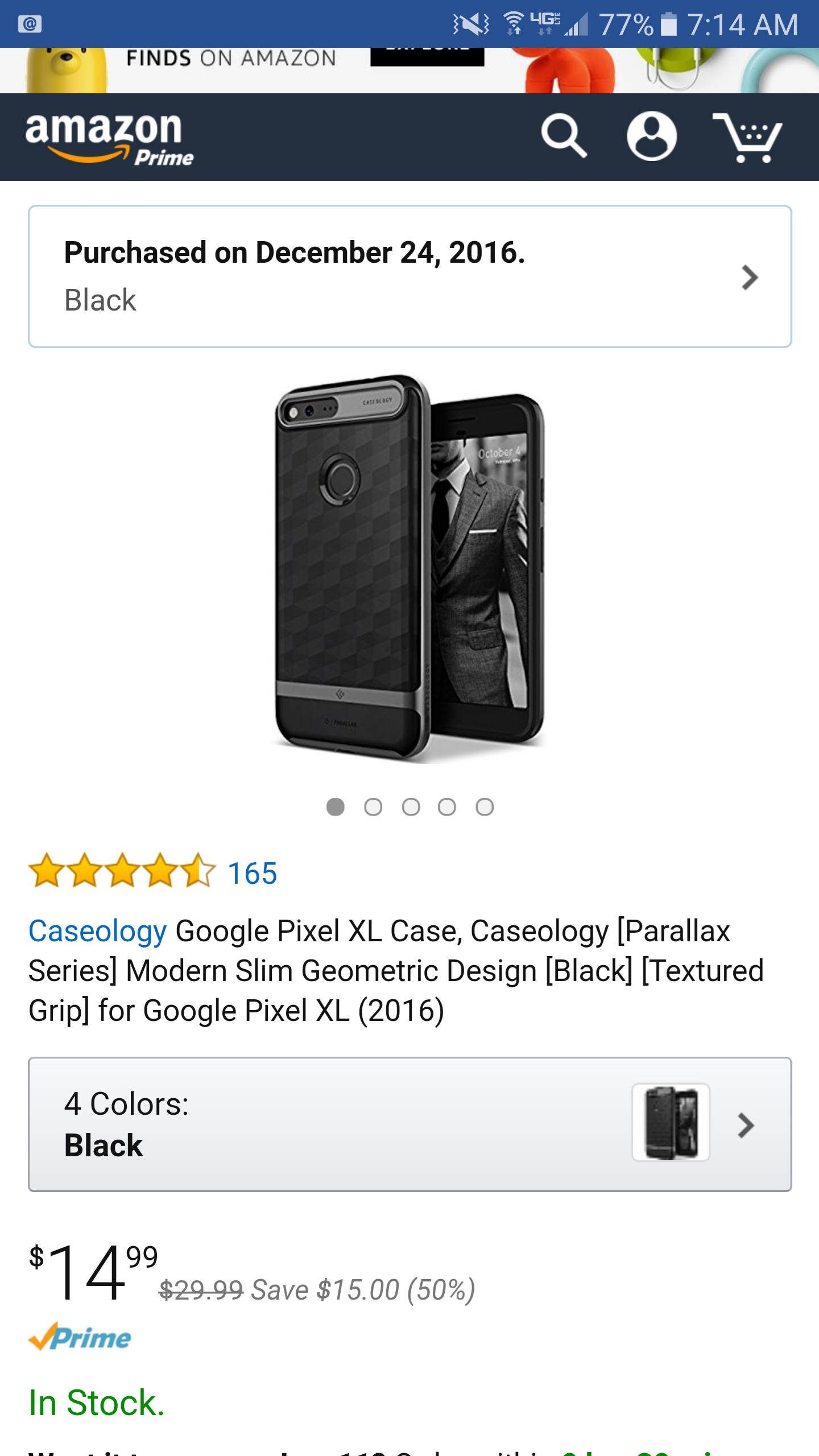The image displays an Amazon store interface on a smartphone screen. At the top of the screen, the Amazon Prime logo is prominently featured, showcasing the word "Amazon" in white with a yellow arrow beneath it. Flanking the top of the screen are three icons on both the left and right: a search button, a profile icon, and a cat icon, all in white against a black background.

Below the icons, the screen transitions to a white background with black text that reads "Purchased on December 24, 2016." Central to the display is a product description for a black device, a Caseology Google Pixel XL case. This product has a rating of 5.5 stars, which are shown in yellow, based on 165 reviews, noted in blue. The brand name "Caseology" is also marked in blue.

The text details the product specifications: "Caseology Parallax Series Modern Slim Geometric Design Black Textured Grip for Google Pixel XL 2016." An image of the sleek, black case is included next to this description. Below the image, there is a note stating that the product comes in four colors, emphasizing the black variant currently displayed.

The pricing information is prominently shown, with the current price listed as $14.99, down from an original price of $29.99, indicating a significant discount. The text "save $15" highlights the 50% savings, all clearly visible. At the bottom, the availability status is confirmed with the familiar Amazon Prime logo, featuring "Prime" in blue and a yellow checkmark, alongside the text "In stock" written in green.